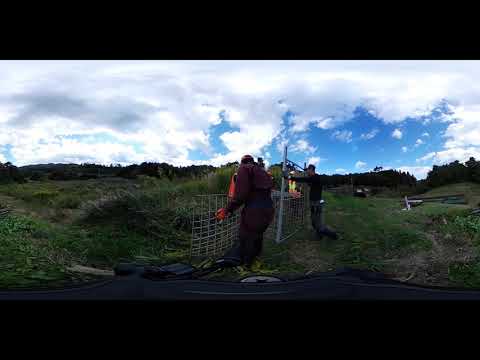The photograph depicts a rural setting with tall grass and a trail to the right. Two light construction workers are featured prominently in the middle of the image. The worker at the center, turned away from the camera, is clad in a dark brown uniform and is handling a waist-height, grey metal fence, seemingly in the process of placing it on the ground. To his right, another worker is seen holding up a taller chain-link fence; this person is dressed in a black long-sleeved shirt and blue pants. Both individuals have their backs to the camera, focused on their tasks. A third person, distinguishable by an orange and yellow safety vest, stands farther in the background, partially obscured by the fence. The backdrop is a stretch of green trees under a mostly cloudy sky with patches of blue. In the foreground, patches of asphalt suggest the proximity of a road. The image has a thick black border on the top and bottom, framing the scene.